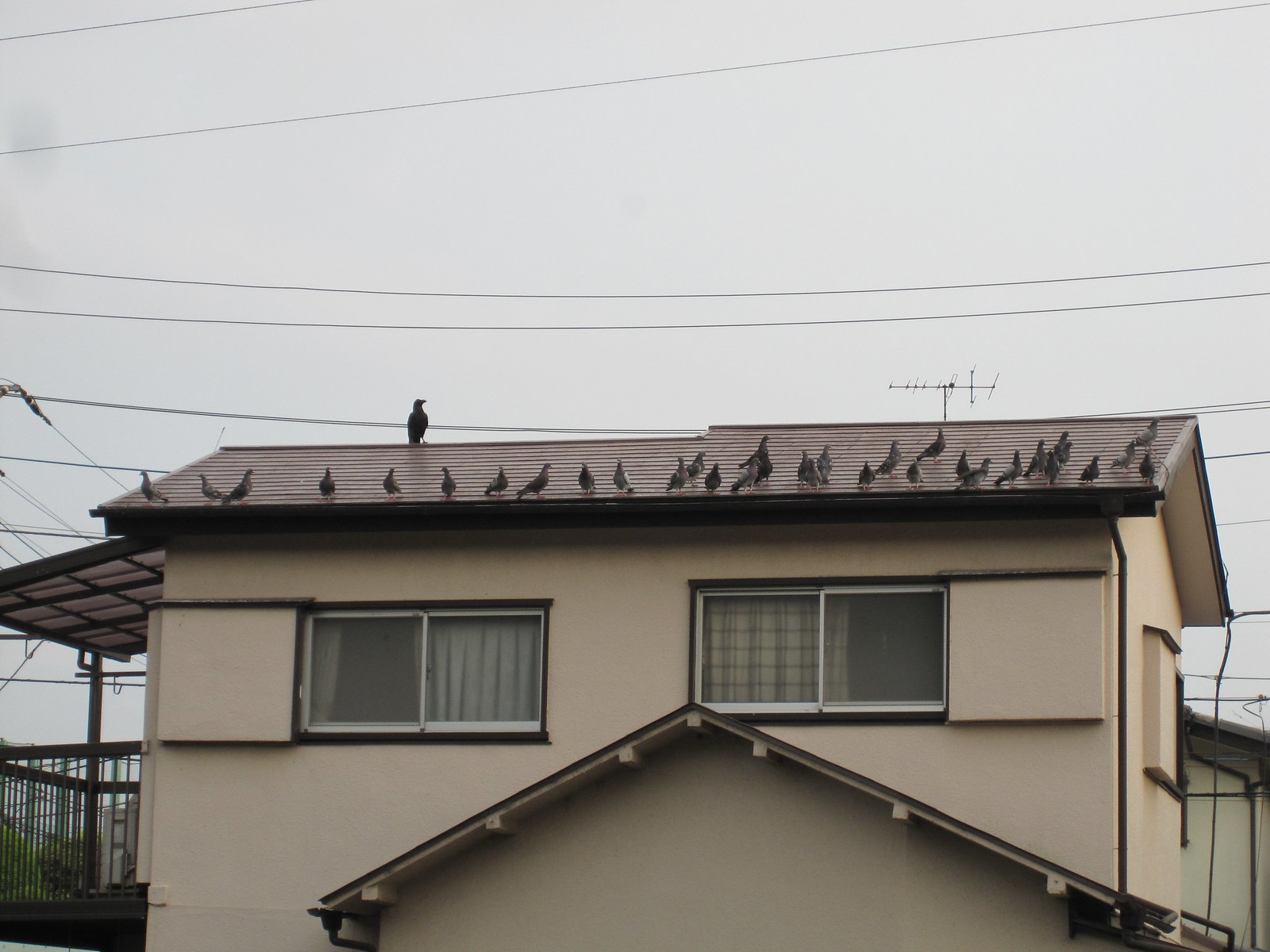The image captures a beige-colored, two-story house with dark brown accents and a shiny, dark brown roof, glistening from the recent rain. The roof features a TV antenna on one side and is crowded with over 20 pigeons and a distinct blackbird, mostly gathered near the edge. The house is equipped with wires descending from the roof to the ground and has visible land lines against a cloudy sky. There is a small front porch and possibly a shed or garage located at the side. Additionally, there are two windows on each side of the house, partially obscured by striped curtains.